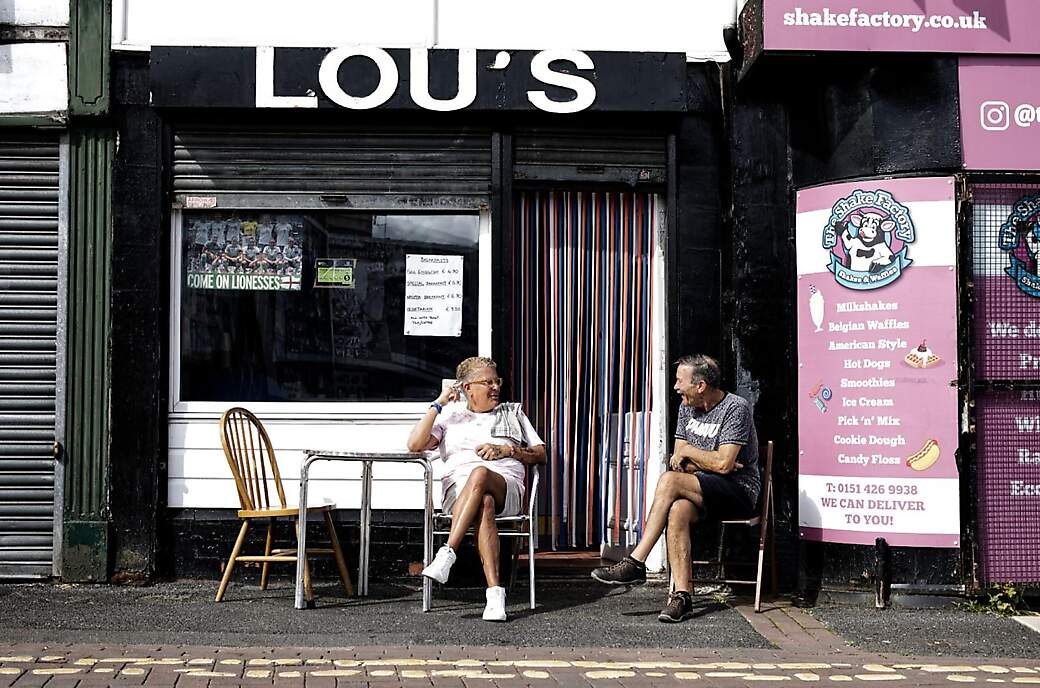The image is a horizontally-oriented, outdoor photograph depicting two elderly individuals seated outside a storefront. The scene unfolds in front of a business with a black awning bearing the name "LOU'S" in white letters. To their right is another establishment named "ShakeFactory.co.uk," marked by a pink banner proclaiming, "We can deliver to you," and offering various items such as milkshakes, Belgian waffles, hot dogs, smoothies, ice cream, cookie dough, and candy floss.

The two individuals, a female on the left and a male on the right, are engaged in a close conversation, their heads bent toward each other. The female is dressed entirely in white – a t-shirt, shorts, and shoes – while the male sports a gray t-shirt with black shorts and dark shoes. They are seated at a single table with three chairs positioned in front of Lou's. The table has an additional wooden chair on the left-hand side. The image seems to be taken from across the street or sidewalk, offering a clear view of both the individuals and the surrounding businesses.